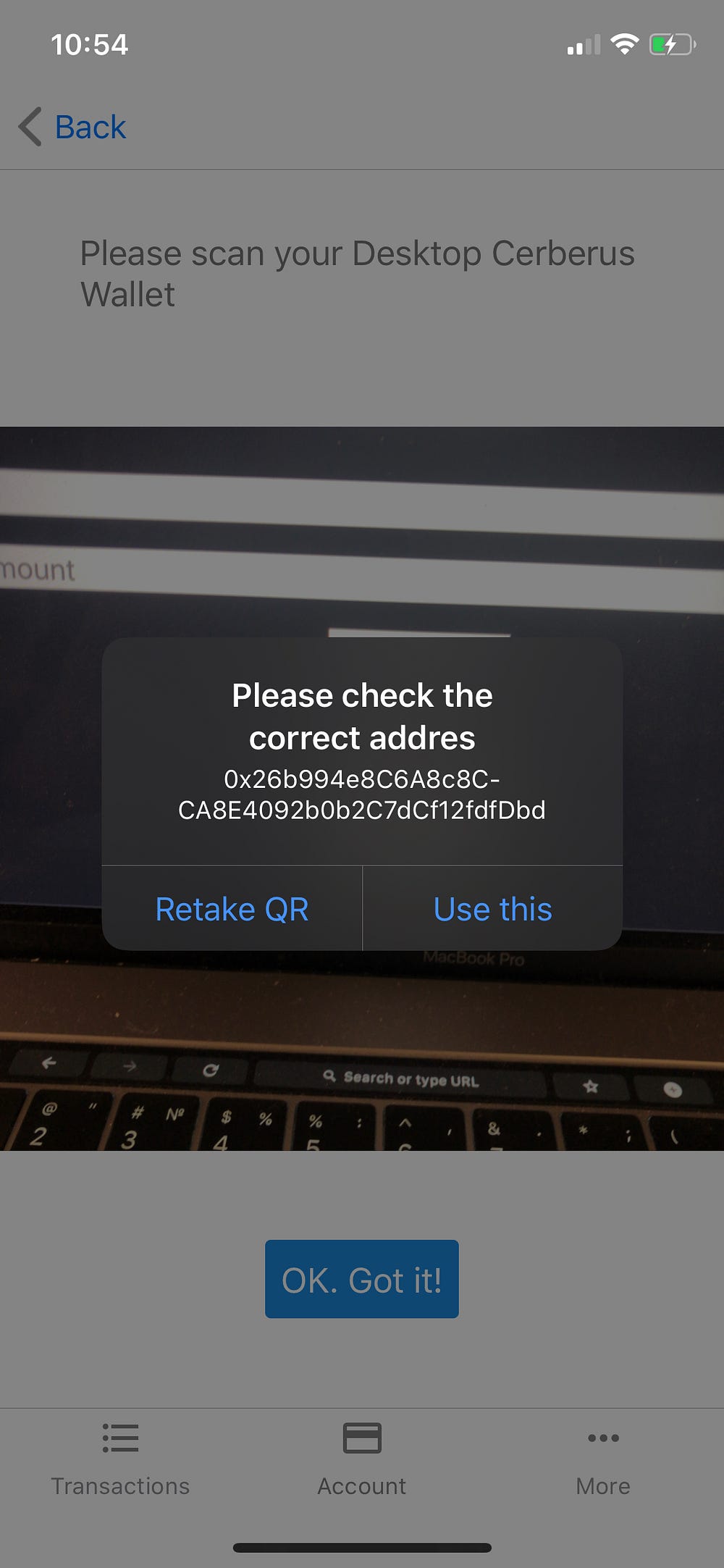The image features a user interface prompt displayed on a mobile device screen. The background of the prompt is black with white text instructing the user to "please check the correct address." Following the instruction is a hexadecimal string "0x26B994E8C6A8C8C-CA8E4092BOB2C7DCF12FDFDBD" that appears to be the address in question. Below this are two options: "retake QR" or "use this".

The surrounding background is predominantly white with blue accents. At the top of the screen, the time reads "10:54," and in the upper right corner are icons for data, Wi-Fi, and a battery charging status. In the center among the user interface elements, an image of a laptop is visible. Below the prompt, the interface offers additional options including "OK, got it" in blue, and tabs labeled "Transactions," "Account," and "More," which are selectable options. Further instructions in gray text prompt the user to "please scan your desktop server as wallet."

Overall, the image appears to show a section of a mobile application or website focused on managing cryptocurrency transactions or similar digital assets.